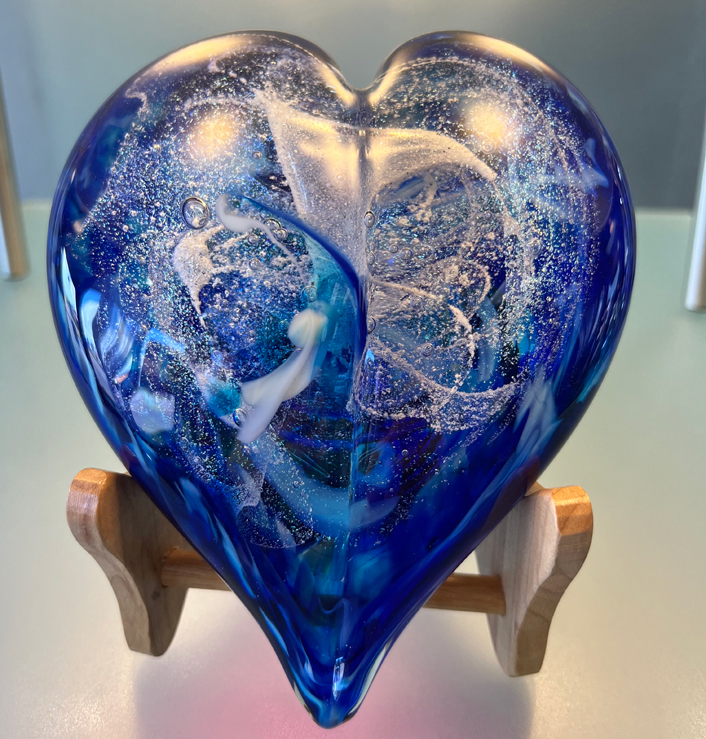This image showcases a close-up photograph of a blown glass heart sculpture perched on a wooden stand. The heart is primarily dark blue, accentuated with swirls of light blue, white, and hints of silver, adding depth and complexity to the piece. Intricately embedded bubbles of varying sizes are visible within the glass, enhancing its textured appearance. The heart is firmly supported in an upright position by a cylindrical rod, attached to light-colored wooden pieces on both sides. These wooden supports are part of a stand positioned on a white surface, with a light gray wall serving as the backdrop. The reflective play of light on the glass heart highlights its artistic craftsmanship and visual depth, though the image provides no explicit scale to determine its actual size.